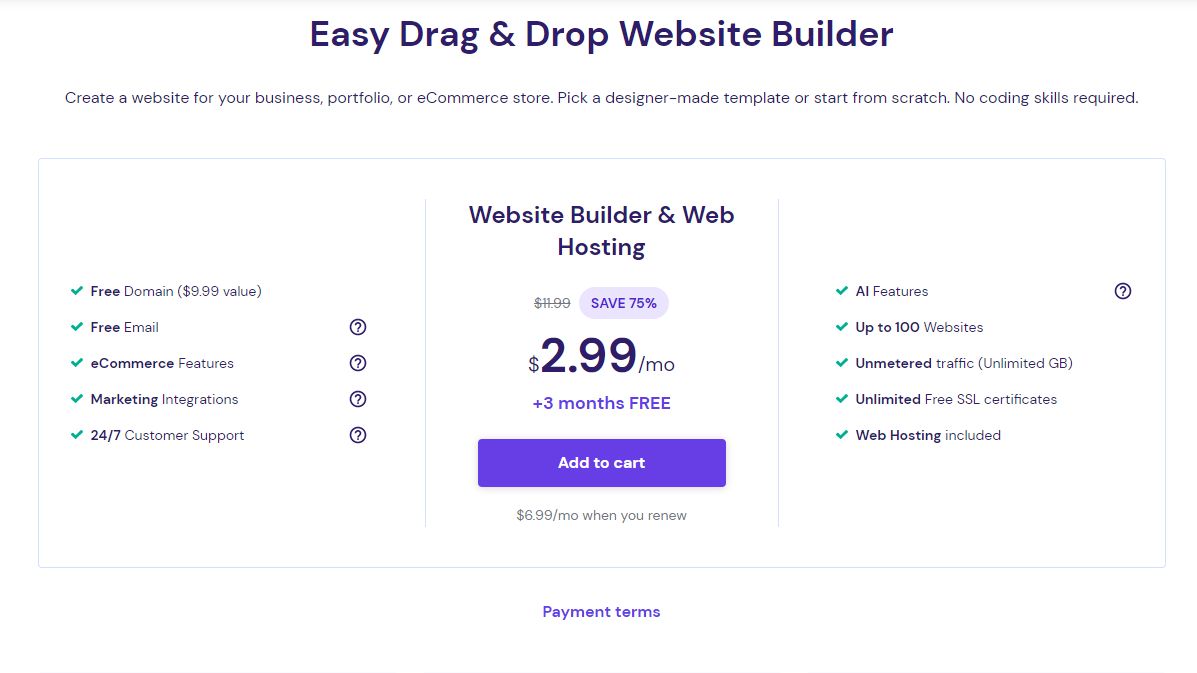**Detailed Caption:**

This is a screenshot of an informational pop-up on a website featuring a sophisticated offer for an easy drag-and-drop website builder. The pop-up sports a clean white background with a subtle gray gradient line at the very top. Dominating the upper section is a headline in bold purple text that reads, "Easy Drag and Drop Website Builder". Directly underneath, in smaller yet distinct text, it states, "Create a website for your business, portfolio, or e-commerce store. Pick a designer-made template or start from scratch. No coding skills required."

Below this introductory text, a rectangular box with a white background outlined by a very thin gray or possibly light blue line appears. This box is divided into three sections by two equally thin lines.

The left-hand column of this box lists key advantages, each accompanied by a green checkmark on the left and most also flanked by a question mark icon on the right for additional information. From top to bottom, the benefits listed are:
- Free domain (with a note indicating a $9.99 value)
- Free email
- E-commerce features
- Marketing integrations
- 24-7 customer support

The center column begins with a bold heading: "Website Builder and Web Hosting". Just beneath this, the original price of $11.99 is visibly crossed out. A purple pill-shaped box next to this displays a "Save 75%" promotion. Below this high-impact announcement, the largest text on the screen prominently showcases the new price of "$2.99 per month", emphasized further by a message in purple text below it, stating, "plus three months free". A large, inviting purple button with white text labeled "Add to Cart" sits directly below. Underneath this button, more gray text notes, "$6.99 per month when you renew".

The right-hand column mirrors the left-hand layout but features distinct offers, with only the first item including a question mark icon for additional details. The items listed from top to bottom are:
- AI features
- Up to 100 websites
- Unmetered traffic (unlimited gigabytes)
- Unlimited free SSL certificates
- Web hosting included